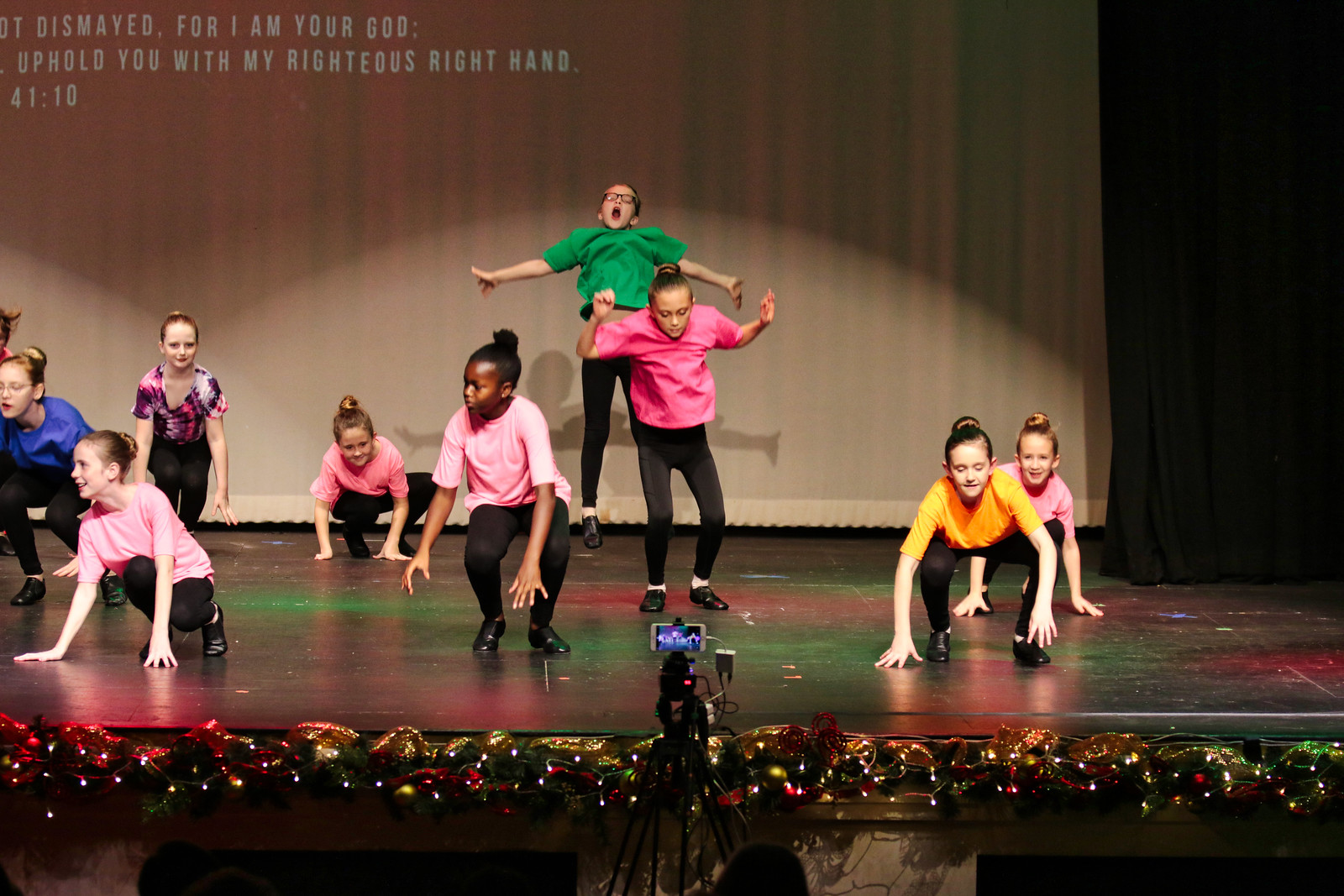The image depicts a lively school concert or Christmas performance featuring a group of children, predominantly girls, aged between seven and ten, on stage. They are dressed in black pants and a variety of colored shirts, including light and dark pink, yellow, green, blue, and a multicolored purple, pink, and white. The scene is festive, with the bottom edge of the stage adorned with Christmas lights, ornaments, and green wreaths intertwined with red ribbons and bow ties. A black tripod with a white smartphone, possibly an iPhone or an Android device, is set up in front, presumably recording the event. The stage backdrop features text from a Bible verse, "Dismayed, for I am your God. Uphold you with my righteous right hand," projected in white. The children appear to be in the midst of a dynamic performance with several jumping and others in positions that suggest they are about to leap. The atmosphere is joyful, with spotlights illuminating the stage and the children smiling and enjoying the moment.